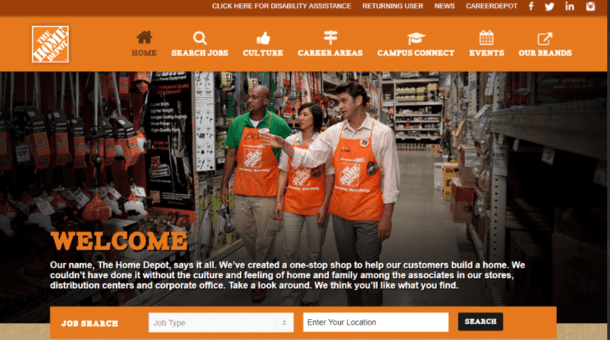This image, sourced from the Home Depot website's welcome page, features a trio of Home Depot employees inside a store, proudly wearing their signature orange aprons. Among them are two men and one woman, representing the diverse workforce of the company. Prominently displayed above is a welcome message reading: "Our name says it all. We've created a one-stop shop to help our customers build a home. We couldn't have done it without the culture and feeling of home and family among the associates in our stores, distribution centers, and corporate office. Take a look around. We think you'll like what you find." Below the text, the page offers several interactive buttons including a job search button, a promotion button, and an events button, alongside sections labeled Career Areas and Culture. A link for disability assistance, marked "Click here for disability assistance," as well as a user account link, further accentuate the welcoming and inclusive environment promoted by Home Depot.